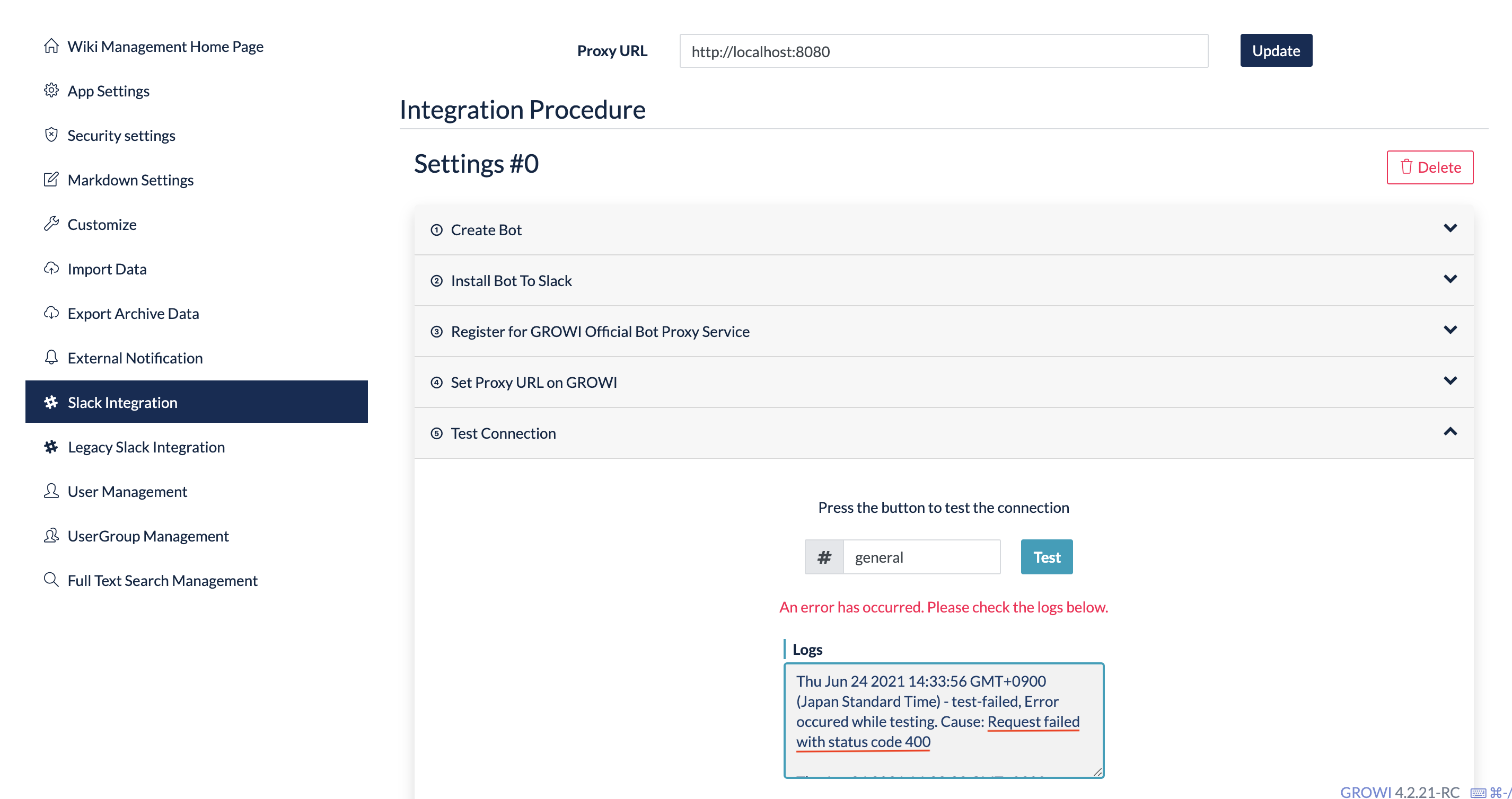Screenshot of a Website Interface Detailing Slack Integration Process:

The screenshot displays a web interface divided into two main sections. 

1. **Left Sidebar Menu**:
   - The menu is set against a white background with blue font.
   - At the top, it reads "Wiki Management Homepage" accompanied by a house icon.
   - Below, there are several menu items, with "Slack integration" being highlighted with a blue rectangle around it.

2. **Main Content Area (Right Side)**:
   - At the top, it displays "Proxy URL" followed by a URL placeholder "localhost:8080" and an "Update" button in blue with white font.
   - Beneath, there is a section labeled "Integration Procedure" accompanied by a "Delete" button.
   - Detailed steps are listed under "Setting Number Zero":
     1. Create Bot
     2. Install Bot to Slack
     3. Register to Grow Official Box Proxy Service
     4. Set Proxy URL and Grow
     5. Test Connection

   - The "Set Proxy URL and Grow" option is expanded, revealing a test connection section.
   - It contains a box prompting to "Press button to test the connection."

3. **Test Connection Section**:
   - The box shows the text "#general test."
   - Below, a red error message indicates: "An error has occurred. Please check the logs below."
   - A fill-in box details the error with the following information:
     - Date: "Thursday, June 24th"
     - Time in Japan Standard Time
     - Error message: "Test failed. Error occurred while testing. Cause request failed with status code 400."

This comprehensive screenshot illustrates the Slack integration process on a webpage, highlighting the current error encountered during testing.